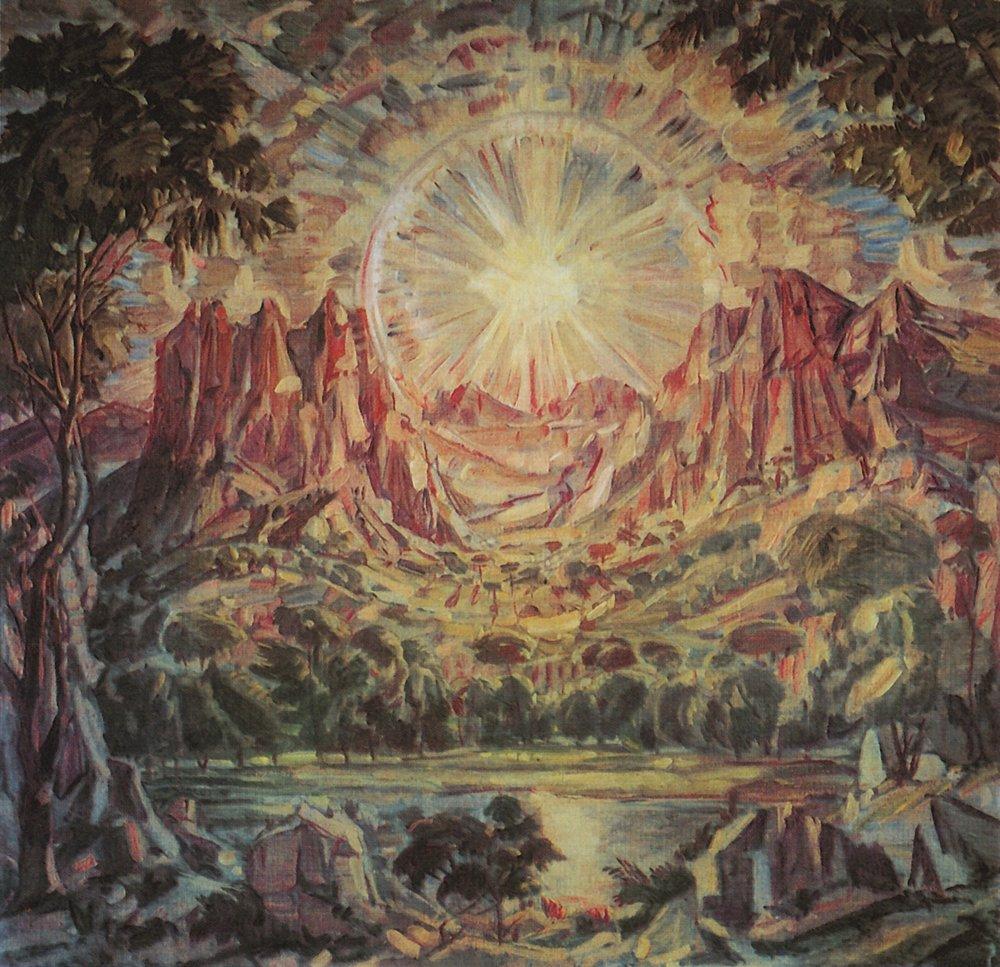The painting is a richly detailed, stylized depiction of a vast and vibrant landscape. The centerpiece of the composition is a radiant yellow orb, presumably the sun, emitting beams of light that illuminate the entire scene. This sun is surrounded by a sky awash in dramatic shades of yellow, blue, and red. Below the sun stretches an array of cliffs and mountains in varying hues of brown and white, seemingly parting to make way for the glowing orb. 

At the base of these cliffs lies a sprawling green valley, dotted with farm fields, clusters of green trees, and quaint houses, creating a sense of rural tranquility. The foreground features a serene blue body of water, which could be a river, pond, or lake, its exact nature beautifully ambiguous. Flanking this water source are lush areas of greenery, complete with dark green trees and scattered fields, adding to the richness of the scene. 

Dominating the left vertical expanse of the painting is a tall tree with dark green leaves, echoing the greenery found throughout the image. The right side also features a similar tree, balancing the composition. Bold and expressive, the painting uses intense colors and patterns—yellows, whites, reds, browns, greens, blues, and even blacks—to create a dynamic yet harmonious tableau that captures both natural beauty and human presence within a lush, almost otherworldly wilderness setting.